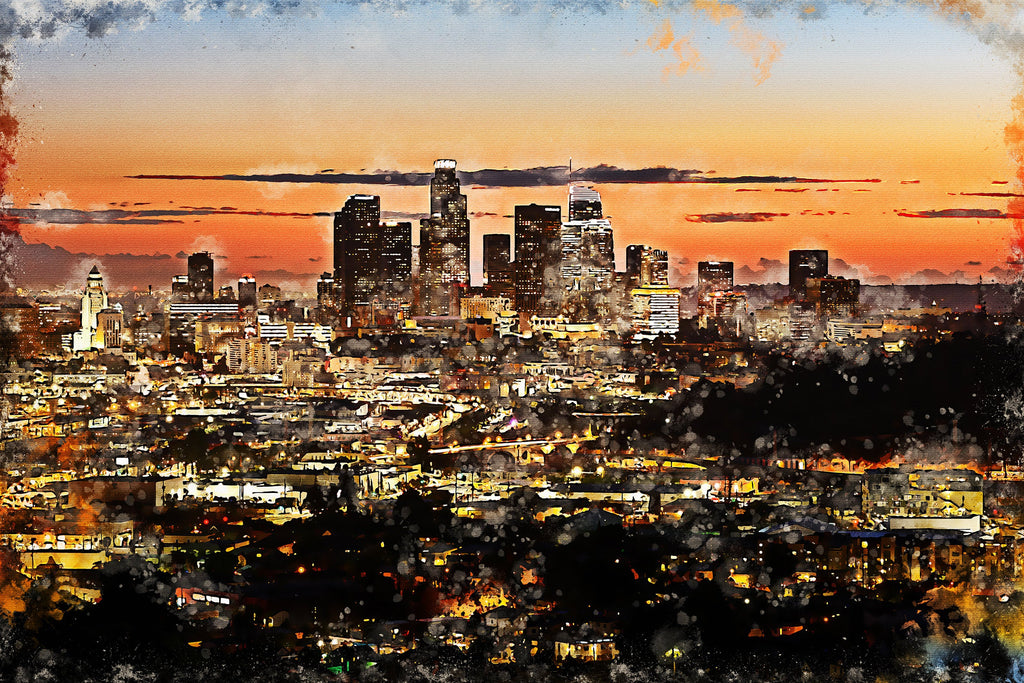The image is a detailed watercolor painting of a sprawling city skyline at deep dusk, capturing the transition from day to night with a vibrant play of colors. The sky, predominantly deep red shifting to orange, culminates in a narrow strip of blue at the very top. Thin horizontal clouds stretch across the sky, enhancing the dramatic effect of the scene.

At the center of the painting, four prominent skyscrapers rise above the city, with the second one from the left standing as the tallest. The cityscape is alight with numerous illuminated buildings, their lights twinkling against the encroaching darkness. Streetlights and stoplights punctuate the scene, hinting at the lively urban activity below. Obscure headlights and the lit-up windows of various homes, businesses, and condominiums contribute to the glowing atmosphere.

The foreground captures a mix of lower buildings and high-rise structures, with scattered trees occasionally breaking the dense cityscape. The edges of the painting blur slightly, giving it an ethereal quality reminiscent of a photograph printed on the front of a postcard. This harmonious blend of light, color, and urban life encapsulates the essence of a bustling city embracing the twilight hour.